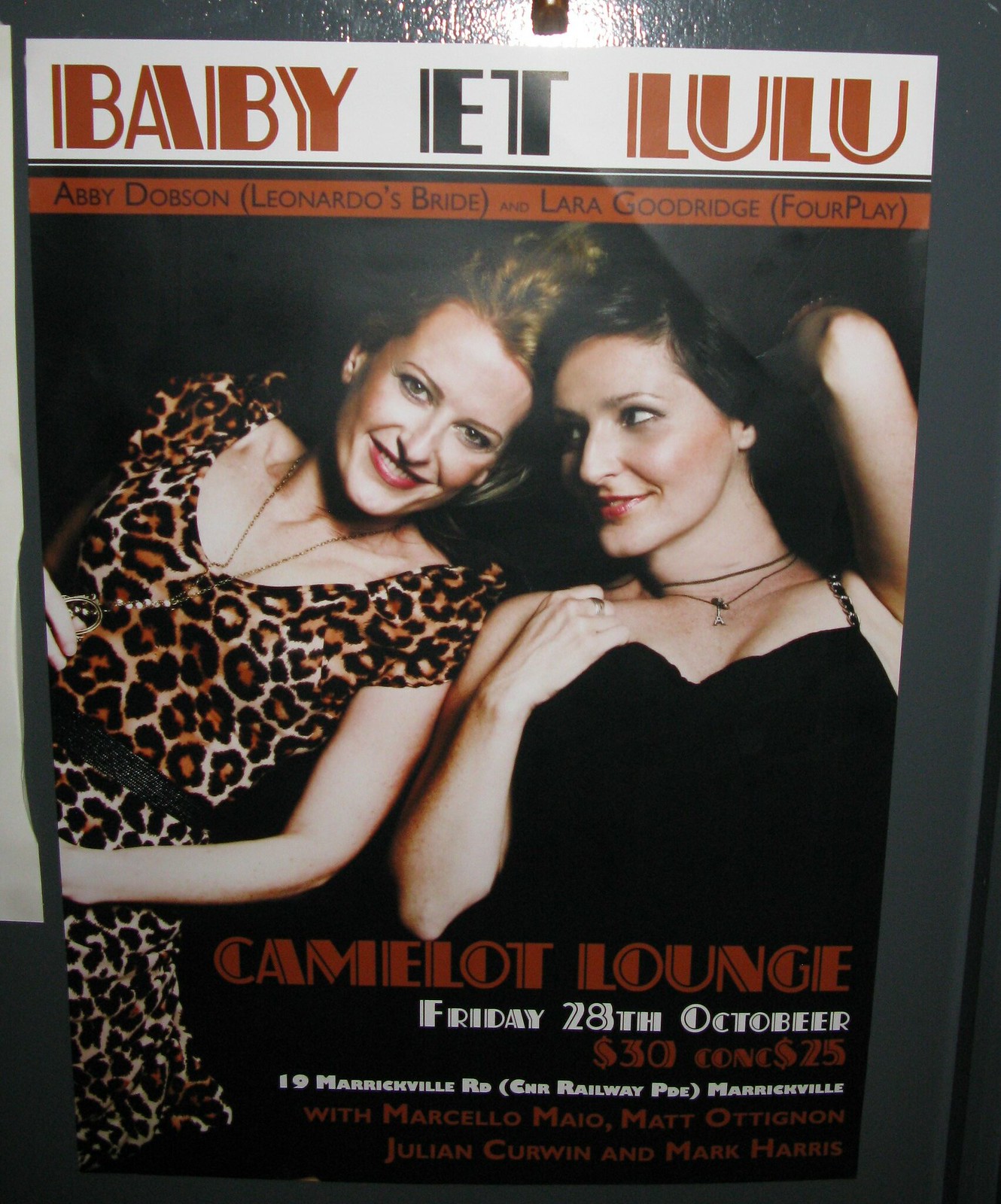This magazine cover or poster features two women, Baby and Lulu, lying on their backs with their heads together, smiling at each other. The woman on the left has blonde hair and is wearing a leopard print dress with a low collar, a black belt, and a necklace. The woman on the right has brown hair and is dressed in a black dress with skinny straps and also wears a necklace. Both appear to be in their late 20s or early 30s.

At the top of the cover, in a white bar with old-school Rococo font, it reads "Baby et Lulu". Below that, in a red bar with black print, the text includes names like "Abby Dobson (Leonardo's Bride)" and "Lara Goodridge (Foreplay)". 

At the bottom of the magazine, in maroon print, it says "Camelot Lounge" and "Friday 28th October". The pricing details "$30" are followed by some additional text that is difficult to read. This promotional material seems to advertise a performance taking place at the Camelot Lounge on the specified date.